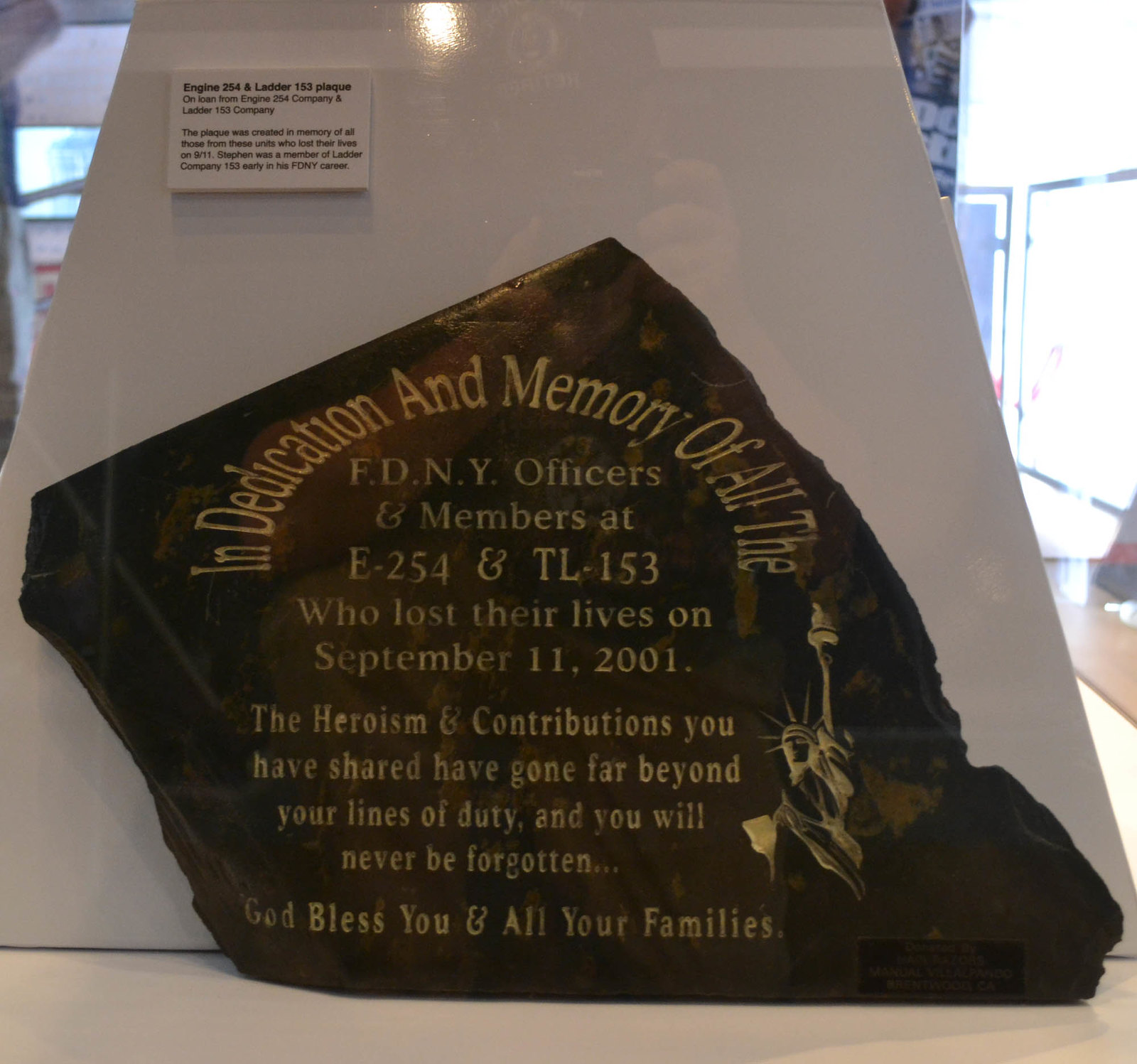This photograph features a beautifully crafted memorial plaque made of dark brown stone, intricately engraved with golden letters. The uniquely shaped plaque, resembling a fragmented rock or an off-centered hexagon, is dedicated to the FDNY officers and members of Engine 254 and Ladder 153 who lost their lives on September 11, 2001. The heartfelt message inscribed in a semicircular fashion reads: "In dedication and memory of all the FDNY officers and members of E-254 and TL-153 who lost their lives on September 11, 2001. The heroism and contributions you have shared have gone far beyond your lines of duty and you will never be forgotten. God bless you and all your families." Carved into the stone is a depiction of the Statue of Liberty, adding to its commemorative significance. A small plaque on the bottom right corner indicates that this memorial is on loan from the respective fire companies. The plaque is currently displayed in a museum or exhibition space, where additional information is provided on nearby labels.